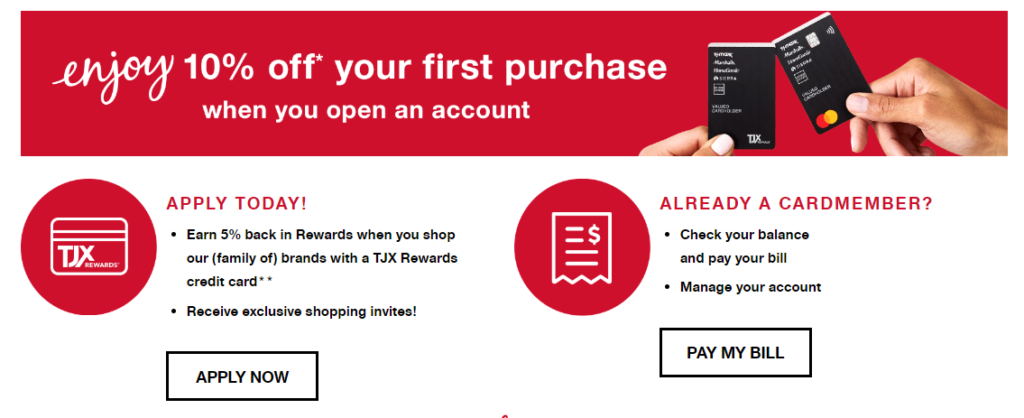At the top of this page, there is a bold red label featuring white text. Below this, a prominent image depicts two hands holding what appear to be credit cards. The white text within this image announces, "Enjoy 10% off your first purchase when you open an account." Directly beneath, detailed information outlines the benefits of applying for the card and includes a prompt urging readers to "Apply Now." Positioned next to this prompt, a red circle with a white border displays the "TJX Rewards" logo. To the right, a section addresses existing card members with options to "Pay My Bill" accompanied by explanatory text. Adjacent to this section, another red circle, seemingly showcasing a printed receipt icon, provides supplementary visuals.